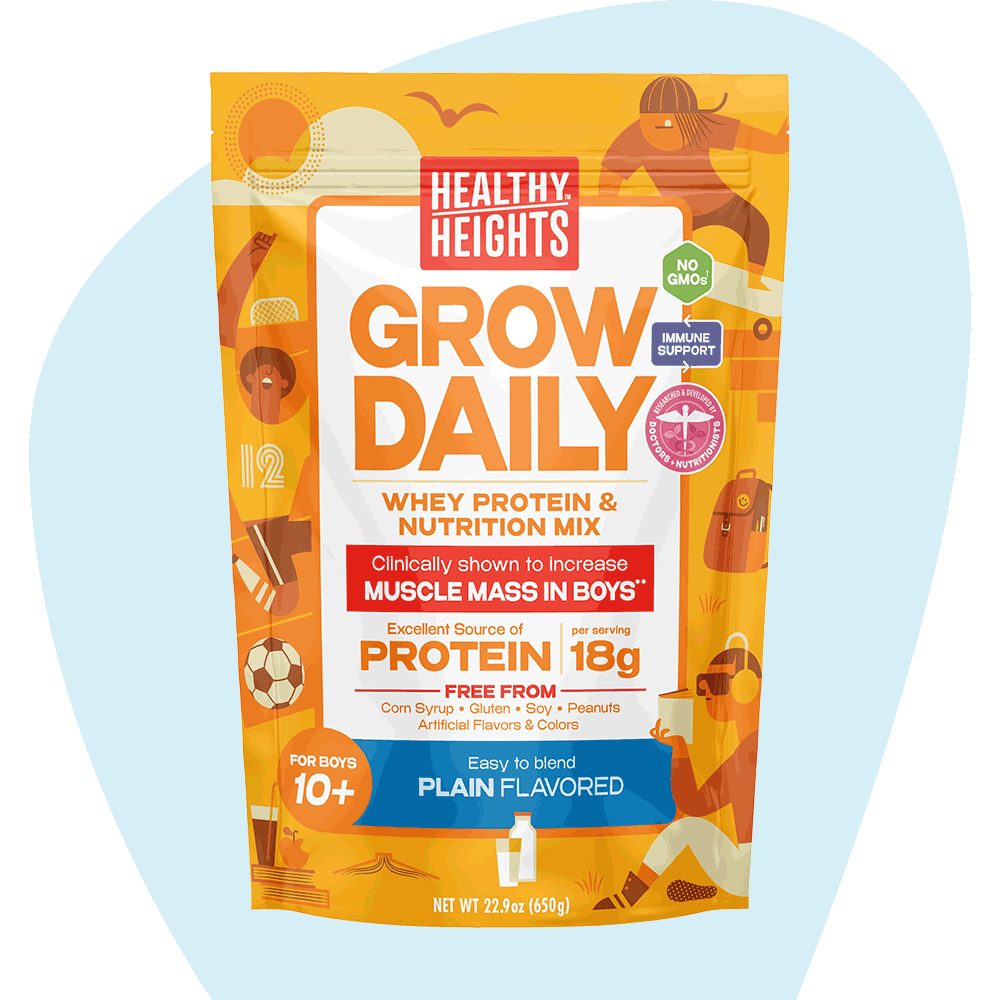The image showcases a prominently featured packaging in the center, with a blue background that is rounded at the top and squared at the bottom. The package itself is primarily yellow and is divided into several text sections. The topmost red box with white text reads "Healthy Heights," followed by an orange text in a white box stating "Grow Daily," which is described as a "Whey Protein and Nutrient Mix." Another red text box mentions that it is "Clinically shown to increase muscle mass in boys." Below this, in an orange text in a white box, it highlights that it's an "Excellent source of protein" providing "18 grams per serving." A red text line followed by orange text details that it is "Free from corn syrup, gluten, soy, peanuts, artificial flavors, and colors." Additionally, a white text in a blue box states "Easy to blend, plain flavored," indicating its suitability "For boys 10 and up." At the bottom, it specifies the net weight as "22.9 ounces" or "650 grams." The packaging is bordered by playful cartoon images of boys engaged in different activities like playing soccer, skateboarding, reading, and listening to headphones. The packaging also promotes that it is free from GMOs and provides immune support.